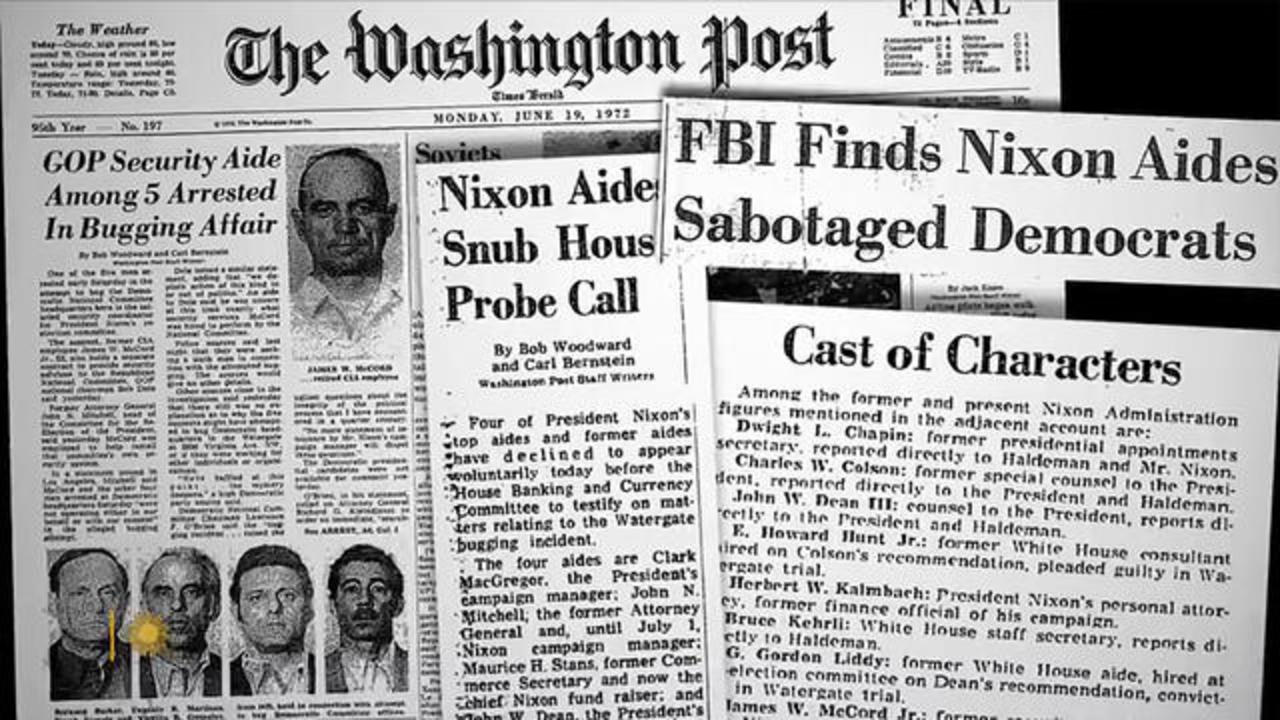This photograph showcases several Washington Post clippings, prominently featuring articles from Monday, June 19, 1972. The clippings focus on the infamous Watergate scandal. The first visible article, headlined "GOP Security Aide Among Five Arrested in Bugging Affair," includes photographs of five men, all with short hair and dressed in collared shirts. The next headline reads "Nixon Aides Snub House Probe Call," followed by another article titled "FBI Finds Nixon Aides Sabotage Democrats." The final headline, "Cast of Characters," lists notable individuals involved in the scandal, providing their names and positions: Dwight Chapin, Charles W. Colson, John W. Dean III, E. Howard Hunt Jr., Herbert W. Kalmbach, Bruce C. Kehrli, G. Gordon Liddy, and James McCord Jr.